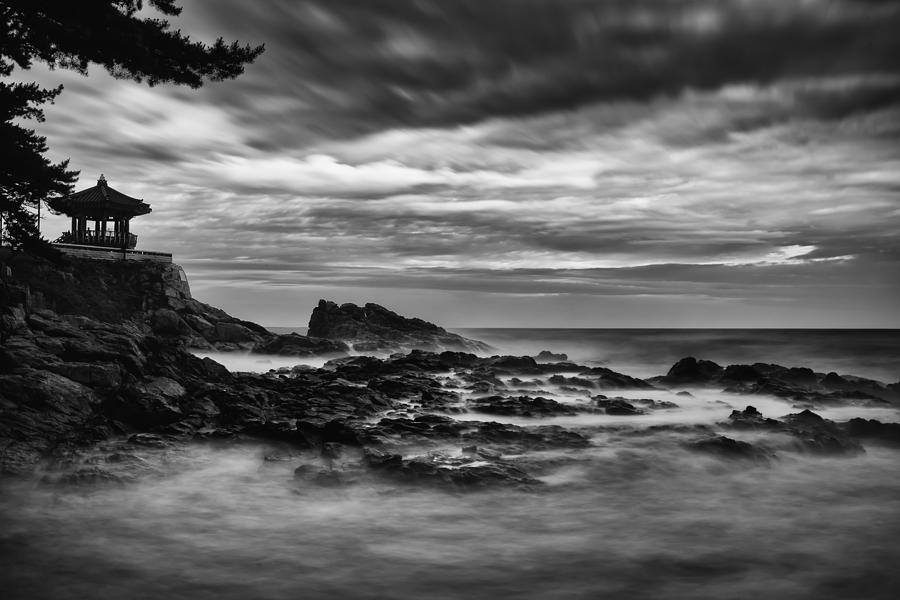The black and white image exudes a moody atmosphere, capturing a serene, fog-laden waterscape under a cloud-filled sky. The clouds vary in intensity, becoming darker and more ominous as they rise, hinting at an impending storm. To the far left, perched on a cliff, stands an Asian-style gazebo or temple, evoking a strong Japanese aesthetic. The gazebo is accompanied by tree branches that extend into view. The rocky shoreline stretches across the middle of the image, with frothy water breaking over the rocks, creating a misty, almost ethereal effect. The smooth water extends beyond the rocks, shrouded in gentle fog. The composition is devoid of people or text, leaving the viewer to immerse themselves fully in the natural and architectural elements that dominate the scene.